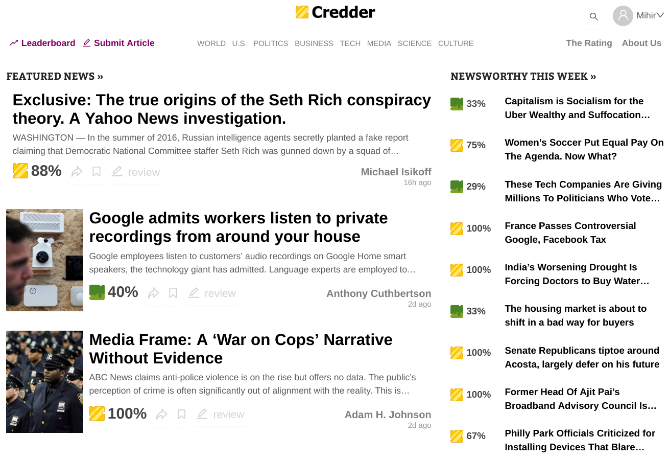Sure, here's a cleaned-up and detailed caption for the image:

---

This screenshot showcases the homepage of the Credder website. At the top center of the page, the Credder logo is prominently displayed in bold black text, accompanied by a square yellow icon to its left. On the far right, there is a gray search icon, a gray circle with a white human silhouette, and the name "MIHIR" with a downward arrow indicating a drop-down menu.

In burgundy text on the upper left, menu options "Leaderboard" and "Submit Article" are visible. Just below the logo, a menu bar featuring various categories is displayed in light gray text, including "World," "US Politics," "Business," "Tech," "Media," "Science," and "Culture." On the far right of this menu, there are additional options labeled "Rating" and "About Us."

The main content area is divided into two columns: a wide column on the left and a narrower one on the right. The left column highlights "Featured News" in bold black text. The first featured article's headline, also in bold black, reads "Exclusive: The True Origins of Seth Rich Conspiracy Theory - a Yahoo News Investigation," which boasts a rating of 88%. Details about the author's name and the posting time are listed to the right of the headline. Beneath, another article titled "Google Admits Workers Listen to Private Recordings from Around Your Home" is displayed, with an accompanying score of 40% in a green icon. Again, the author's name and posting time are shown on the right side.

The final featured headline, "Media Frame a 'War on Cops' Narrative Without Evidence," appears in bold black text along with a picture on the left. This article has an orange icon indicating a 100% rating.

On the right-hand side, the column is labeled "Newsworthy This Week" in bold text. A vertical series of headlines with percentage ratings follows, each identified with yellow and green icons on the left side.

---

This caption provides a clear, comprehensive overview of the webpage's layout and content.